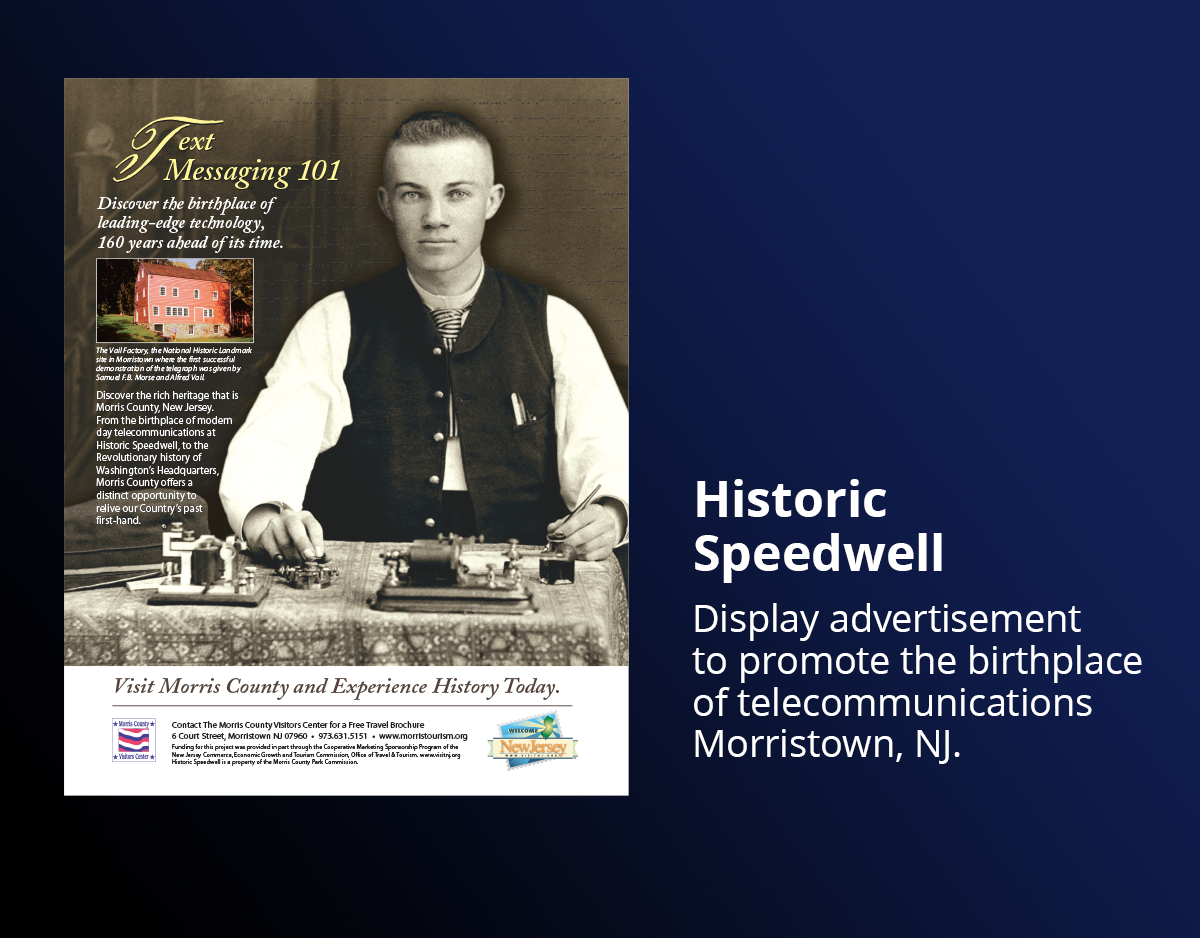This image showcases a landscape-oriented presentation slide designed for a historical education setting, focusing on the origins of telecommunications. The slide's background is a gradient transitioning from dark blue to black. On the left side, there is a black-and-white, portrait-oriented photograph of a man with a short haircut, dressed in vintage attire, sitting at a desk equipped with old telegraph and telex machines, suggesting a bygone era. Above the photograph, in cream-colored text, the headline reads, "Text Messaging 101: Discover the Birthplace of Leading-Edge Technology, 160 Years Ahead of Its Time." Below this image, there's a color photograph of a building, accompanied by text that states, "Visit Morris County and Experience History Today," alongside some logos and flags. On the right side of the slide, in white text on a dark blue-to-black gradient, is the title "Historic Speedwell" in bold, followed by the subtitle, "Display Advertisement to Promote the Birthplace of Telecommunications, Morristown, New Jersey." The entire caption highlights colors such as blue, gray, dark gray, brown, white, black, pink, and green, emphasizing the blend of historical significance and modern presentation techniques.